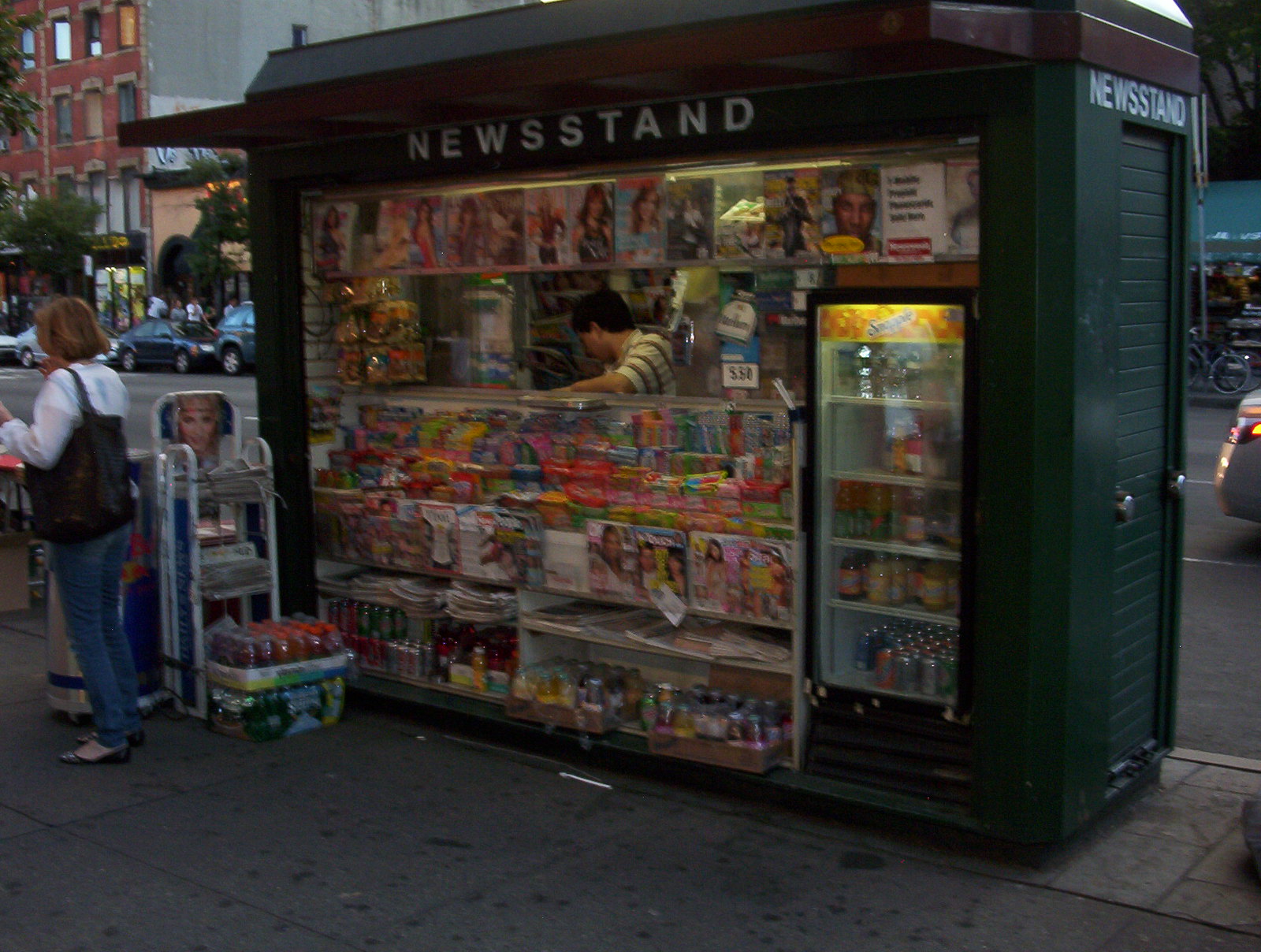The image depicts a green rectangular newsstand on the sidewalk of a busy street, possibly in New York City. The newsstand, detailed with a brown roof and brown trim, bears the word "newsstand" in white font on both the front and right side. A man dressed in a green and tan striped shirt works behind the counter. To the left of the newsstand, a woman with honey brown hair, wearing flat shoes, blue jeans, a long sleeve white blouse, and a black shoulder tote bag, is seen browsing. Beside her is a newspaper rack showcasing a picture of a blonde woman's head. In the background, cars are parked along the far end of the street. The newsstand is stocked with various magazines, candies, and sodas, including a Red Bull container, bottles of Gatorade, a Snapple cooler filled with assorted Snapple, Coke cans, and a Marlboro sign indicating cigarette sales.